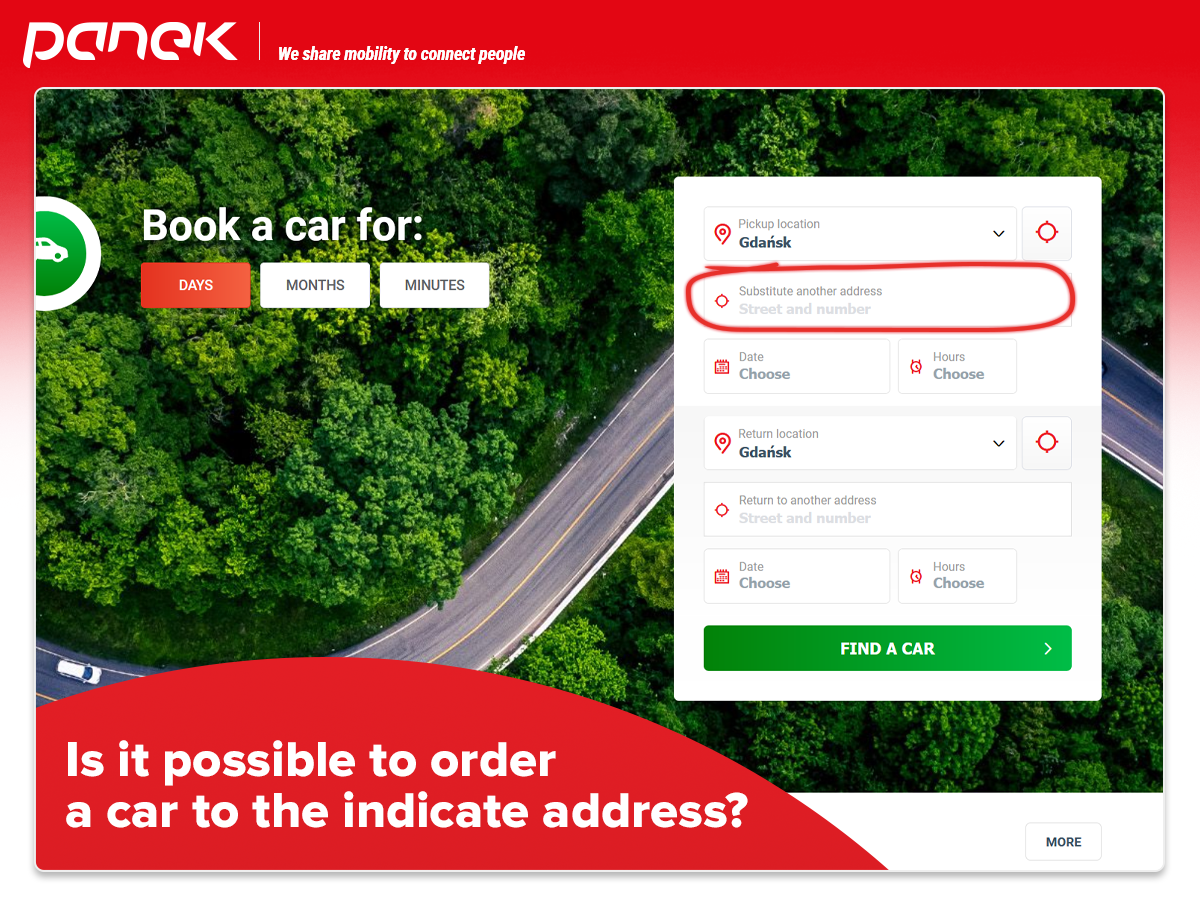The image depicts a web page for a car rental service named "Panek." At the top of the page is a logo, which is bordered in red and displays the company name "Panek" in white text. Adjacent to the logo is the slogan, "We Share Mobility to Connect People." Below the header, there's an aerial photograph showing a scenic view of trees flanking a road or highway. Overlaying this image are options for booking a car, with buttons labeled "days," "months," and "minutes" to specify the rental duration. To the right of the photograph is a pop-up menu with fields for "Pickup Location," "Substitute Another Address," "Date," and "Hours." There are also drop-down menus for "Return Location" and "Return to Another Address," along with additional fields for specifying the "Date" and "Hours" of return. At the bottom of this menu is a prominent green button labeled "Find a Car."